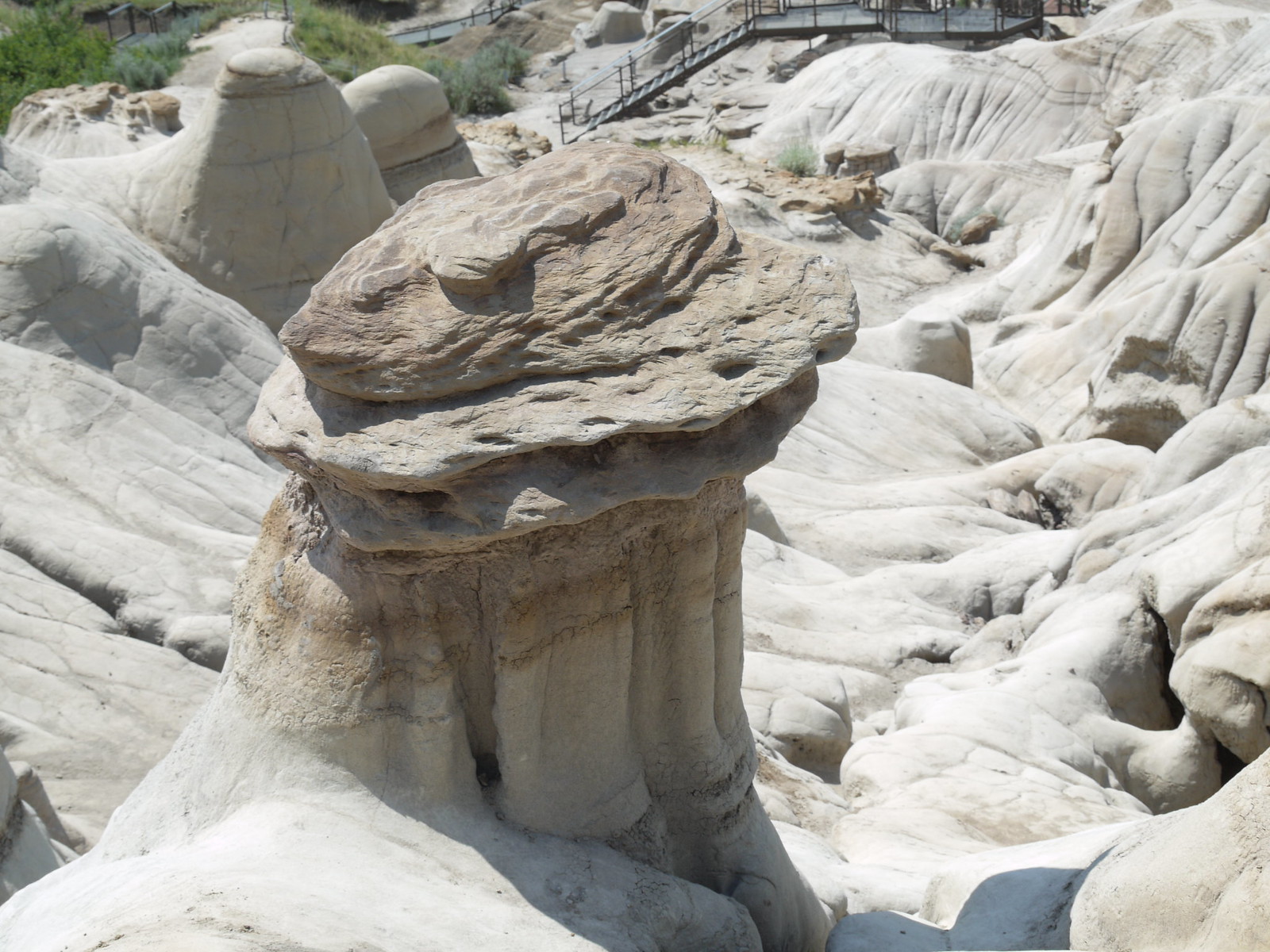This color photograph, taken outdoors during the daytime in a desert setting, captures a range of earthy tones including shades of brown, grey, and beige, with touches of green. The photo depicts a very dry, stony landscape with minimal vegetation, except for a couple of bushes or small trees in the upper left corner. Toward the center of the image, steps lead up to what appears to be a building, possibly a cabin. The natural rock formations dominate the scene, featuring smooth, almost volcanic surfaces and intricate geometric designs shaped by water erosion over the years. These formations include lines that mark sediment layers, swooping riverbed-like structures, and protruding shapes that resemble tiny hills or mushrooms.